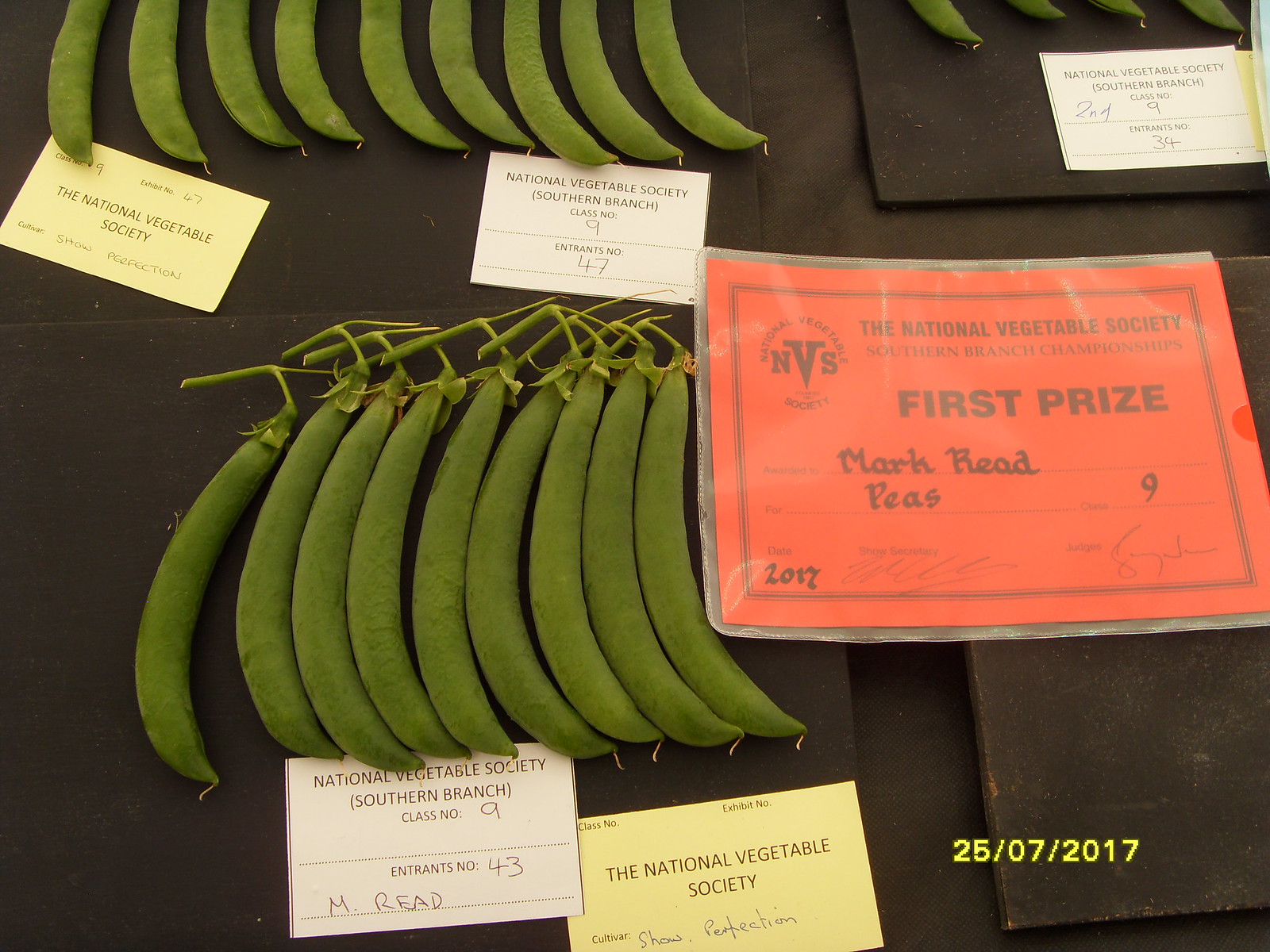This detailed photograph captures an award-winning display of pea pods from the National Vegetable Society, taken on July 25, 2017. The image presents an overhead flat lay of vibrant green pea pods meticulously aligned in a horizontal row across a dark brown surface. Each pea pod, about four to five inches long, faces right with their stems slightly bent to the left, highlighting the grower's professional skill. 

An orange certificate to the right of the peas bears the emblem of the National Vegetable Society and the handwritten name "Mark Read," denoting his first prize win for the peas category. Above the main row, another partial row of pea pods can be seen, accompanied by blurred index cards. Additionally, at the bottom center of the image, a white index card with printed and handwritten details indicates "National Vegetable Society (Southern Branch)," class number "9," and reiterates "M. Read" as the contestant. Below this card is a yellow one, similarly branded with the National Vegetable Society's logo and more handwritten text.

This award-winning shot not only showcases the impressive quality of the pea pods but also emphasizes the precision and care taken in displaying these prize vegetables.